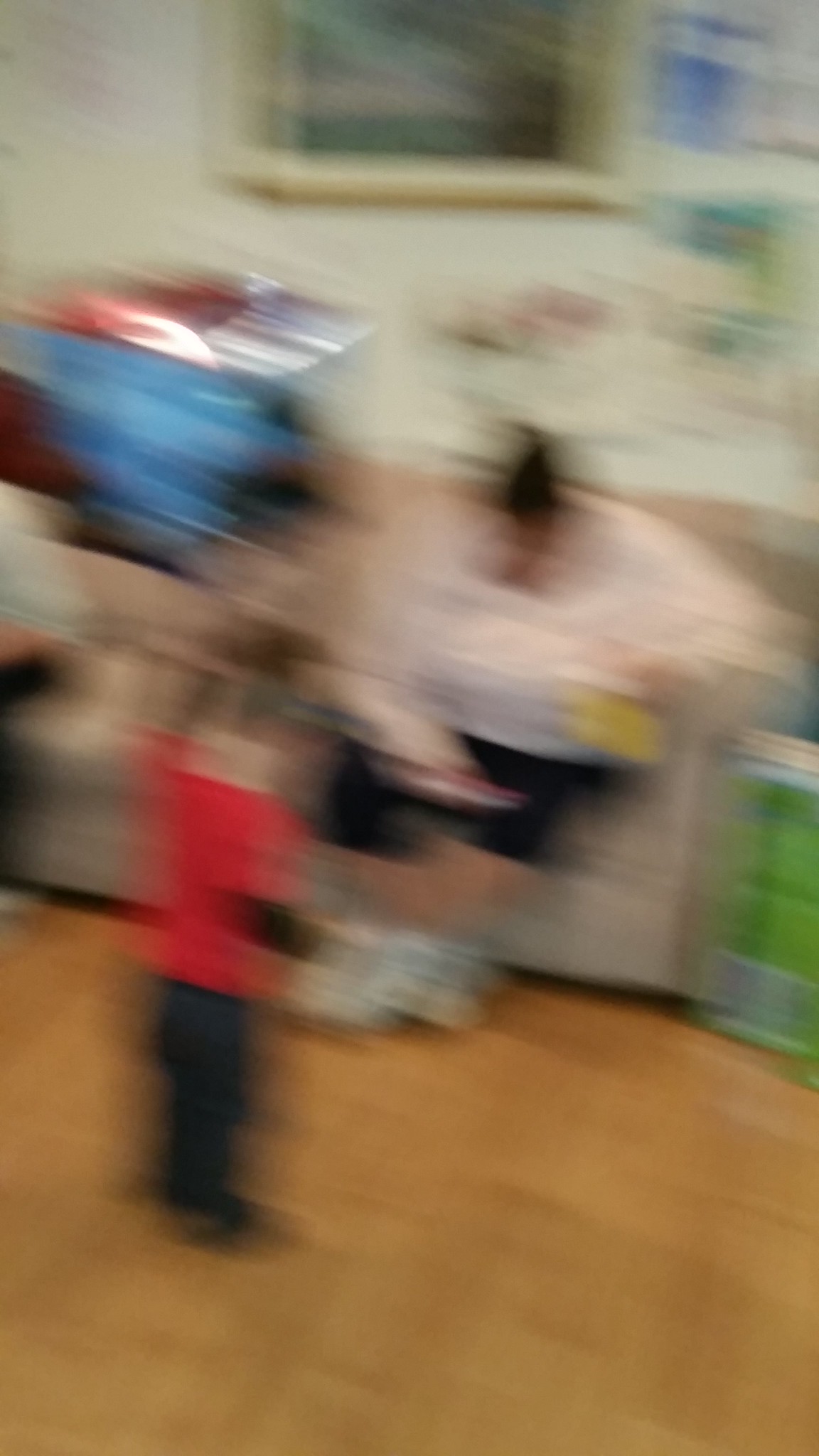A blurry, motion-captured image depicts a chaotic scene in a dimly lit room with a wooden floor. In the foreground, a child, dressed in black pants and a red shirt, is barely discernible, possibly due to movement. Another figure, potentially plus-sized, sits on a couch or chair, clad in black shorts and a white shirt. The background features a wall adorned with either artwork or a window, though it's unclear due to the blurriness. Shades of blue streak across the image, suggesting rapid movement, but their source remains ambiguous. The photograph conveys a sense of dynamic activities and lacks any visible text.